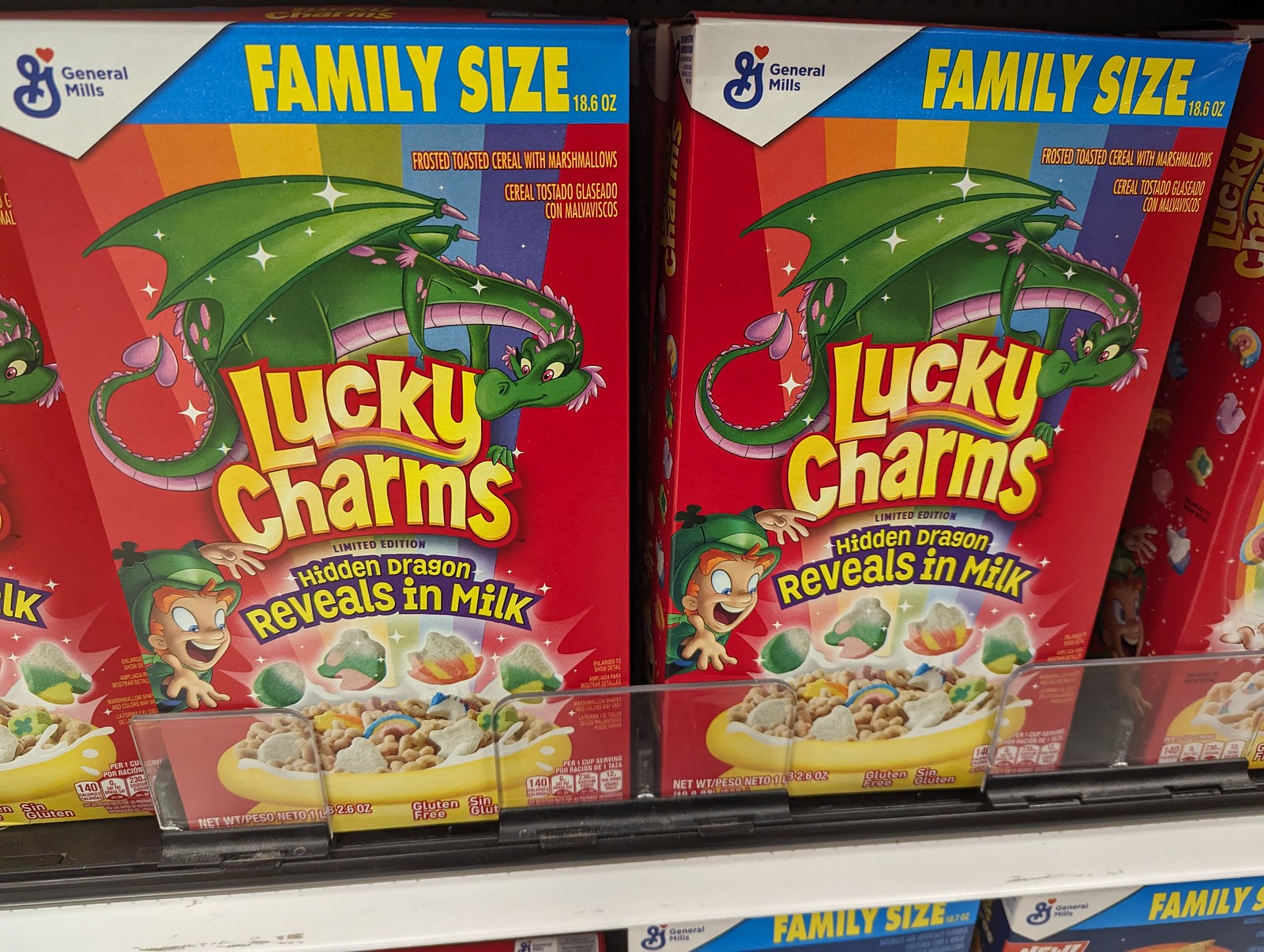The image captures neatly organized supermarket shelves displaying multiple family-sized boxes of Lucky Charms cereal. The main focus is on two prominent boxes positioned side by side, featuring the distinctive branding and vibrant colors typical of Lucky Charms. The shelves, constructed from a white metal frame and equipped with a black tray, host these eye-catching cereal boxes.

Each box prominently displays the General Mills logo in the upper left-hand corner, a blue stylized "G" inside a white box, accompanied by a red heart, signifying a General Mills product. To the right of this logo, the phrase "Family Size" is emblazoned in bright yellow letters, alongside the weight specification of 18.6 ounces.

The iconic Lucky Charms logo is rendered in its classic yellow lettering, and a captivating green dragon swirls around it, indicating a special edition. The text “Hidden Dragon Reveals in Milk” is situated beneath the main logo, hinting at the magical experience awaiting consumers. Additionally, Lucky the leprechaun is depicted to the left of the logo, animatedly raising his hands as if conjuring marshmallows into the air, enhancing the whimsical feel. A bowl of cereal with floating marshmallows further adds to the lively design.

Adjacent rows of boxes and more Lucky Charms on both the top and bottom shelves suggest a well-stocked display, emphasizing the product's availability. The scene captures the vibrant and enchanting appeal of Lucky Charms cereal in a typical grocery store setting.